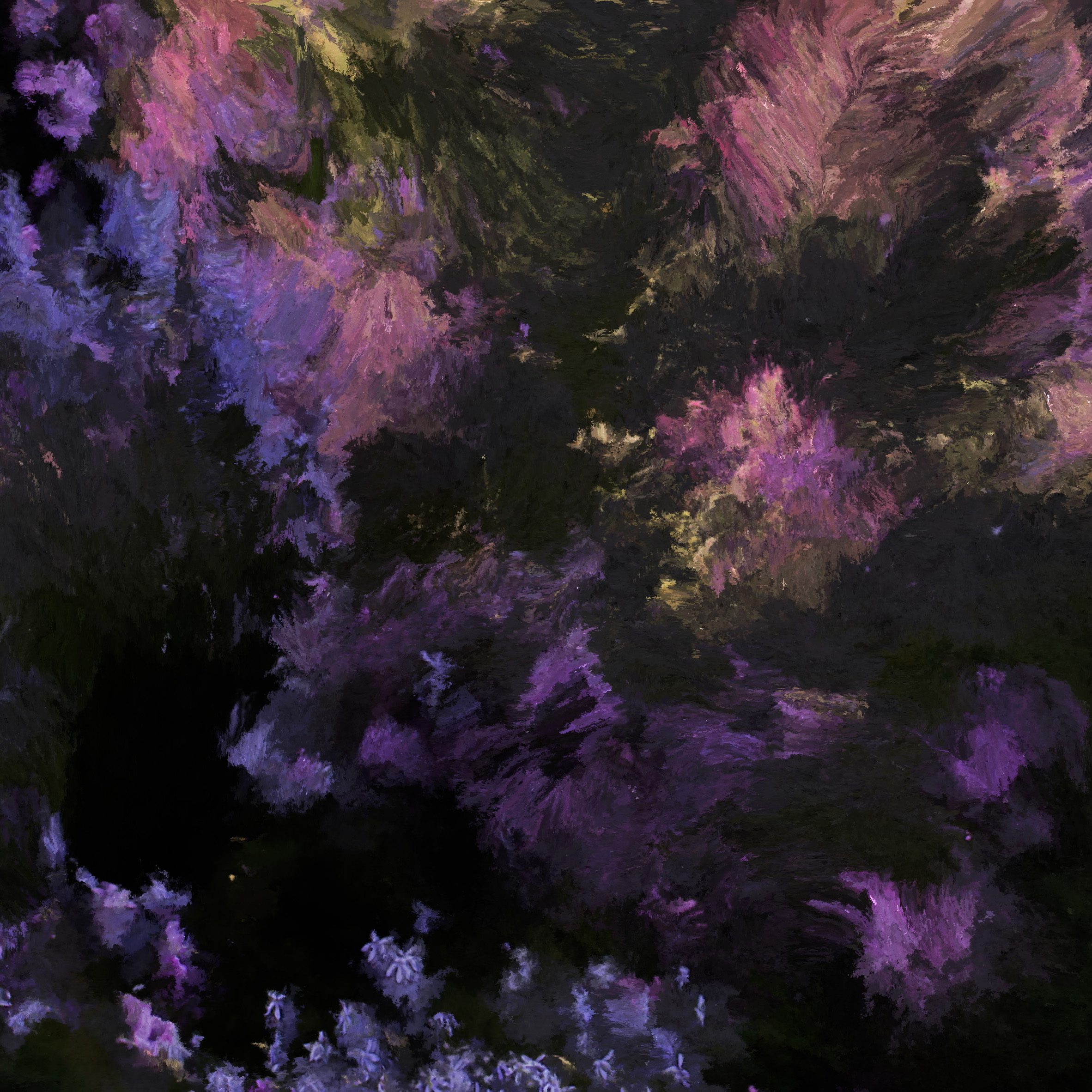This image is a painting with no text, featuring a predominantly black and purple color palette. The background is mostly black, with splashes and strokes of color throughout. The bottom left corner is almost entirely black, punctuated by small splashes of purple and what appear to be white flowers on purple plants. The bottom edge of the painting seems to be adorned with purple flowers, blending in with the black background. The bottom right corner continues this theme, with mostly black and subtle purple splotches. 

In the middle section, there are black splotches interspersed with a notable splotch of purple and green toward the right edge. At the top left corner, light purple hues possibly representing flowers are visible, contrasted by dark black elements. The top right corner features more light purple alongside black splotches. 

A unique feature is a hint of yellowish color near the top center, slightly to the left, adding a sense of light shining through the otherwise dark composition. The strokes of color become broader and more pronounced towards the top, transitioning to smaller, more directed strokes that resemble flower petals as they move downward. The painting has an abstract quality, making it challenging to distinguish specific elements, but the overall impression suggests a dynamic interaction between the floral forms and the stark, dark background.